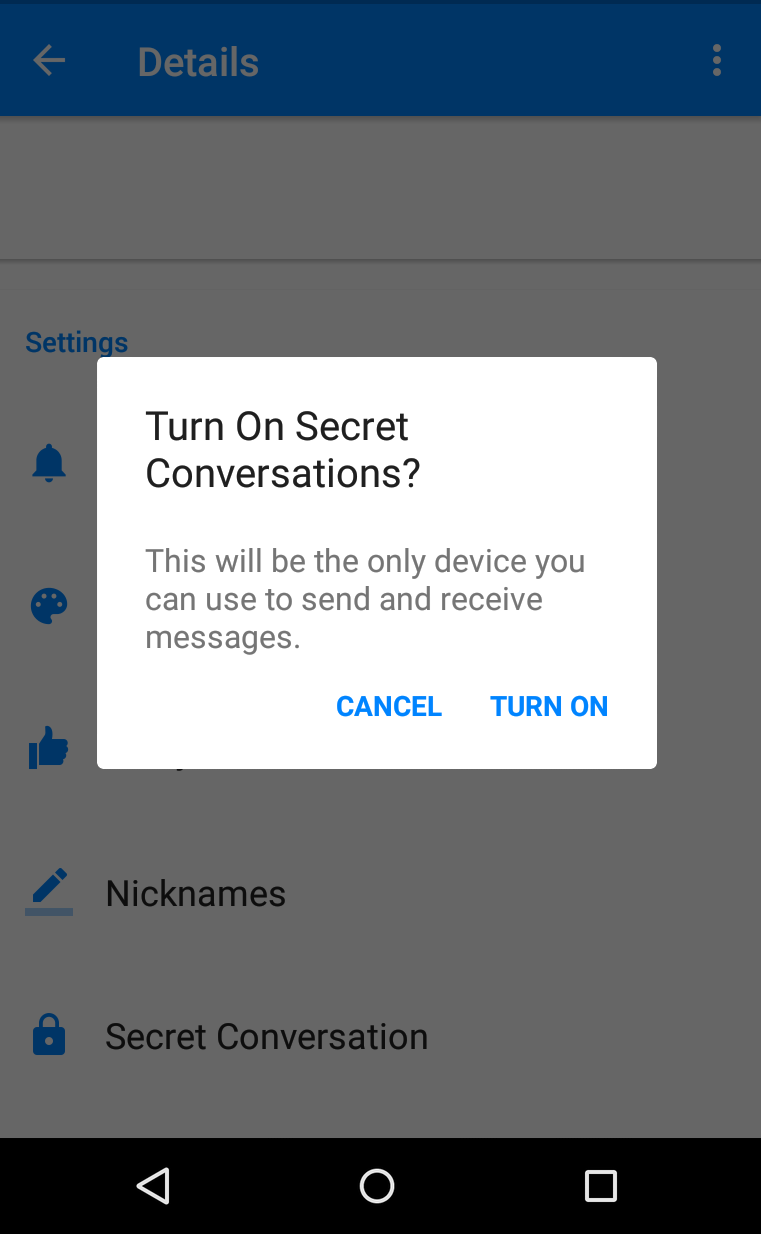The image is a screenshot showcasing a notification-like pop-up box. At the top of this box, aligned to the left, is the bold heading, "Turn on secret conversations." Below this heading, the text provides a cautionary message: "This will be the only device you can use to send and receive messages." At the bottom right corner of the box, there are two buttons: the one on the left is labeled "Cancel" in bold blue letters, while the button to the right also in bold blue letters says, "Turn on." The background outside of the pop-up suggests that the user is currently in a settings area of a webpage.